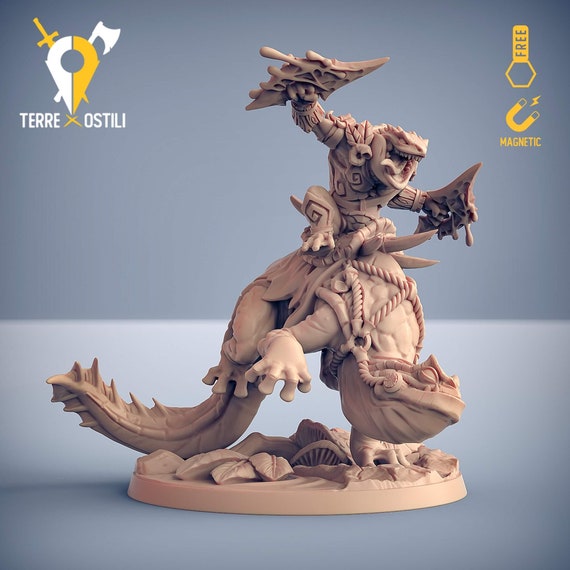This is a detailed depiction of a computer-generated figurine, showcasing a battle-ready toad-like warrior mounted atop a large lizard-like creature. The toad-like figure, resembling a warrior, is equipped with two war axes and adorned with armor. The lizard beneath it is harnessed with ropes and a saddle, suggesting it has been tamed by the warrior above. The scene is set against a dual-tone gray background with the top part darker than the bottom. The figurine rests on a blue surface, contrasted by a darker blue background. Notably, the upper left corner features a yellow sword and axe icon accompanied by the white text "Terra Asteli" with a yellow X between the words. Additionally, the upper right corner shows a pentagon with a yellow rectangle and a yellow magnet with a lightning bolt, labeled "Magnet". This intricately designed piece appears to be more of a shelf display rather than a toy, capturing the essence of a fantastical battle scene.